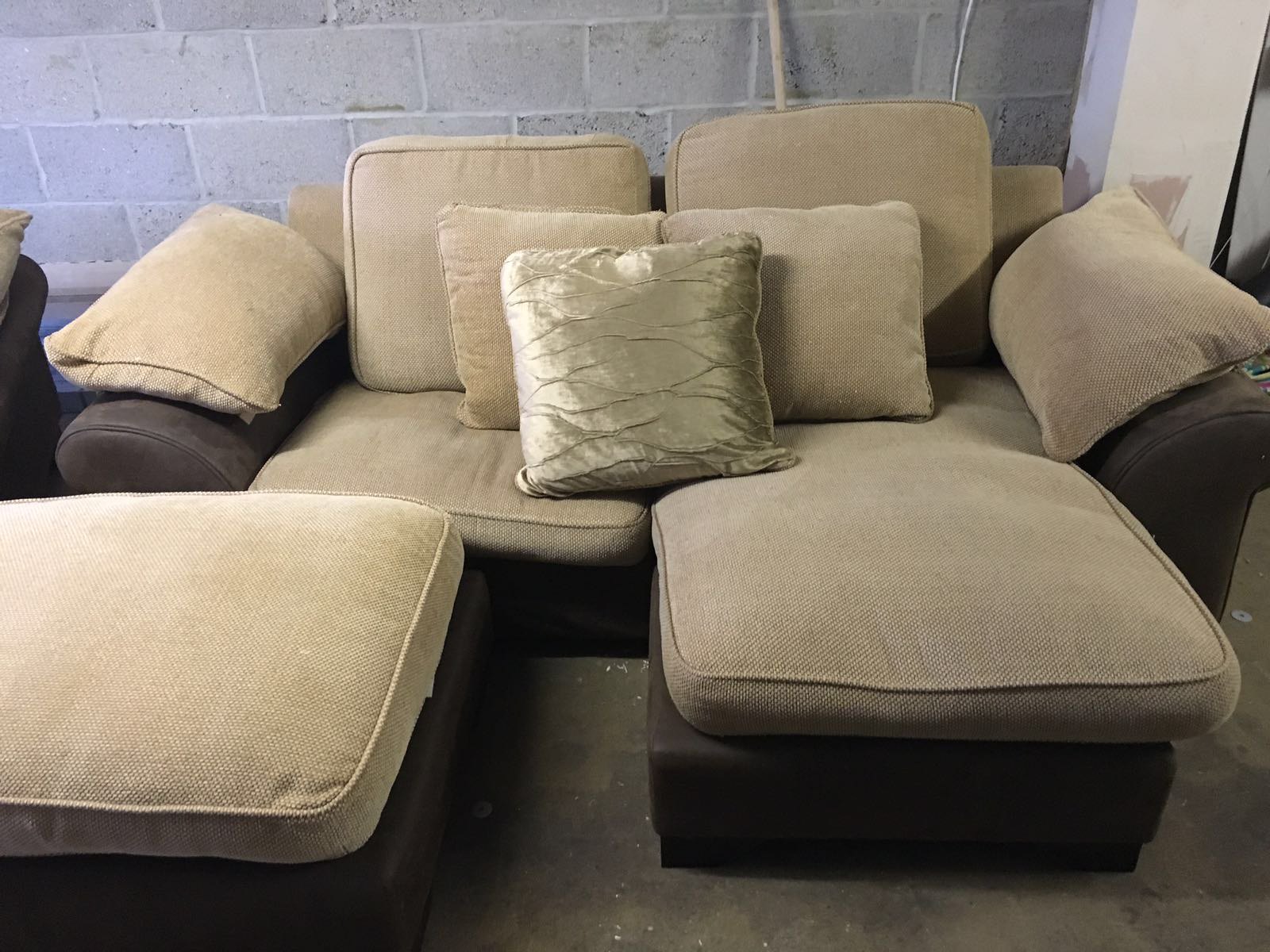This photograph features an old, beige couch with a combination of canvas and darker brown materials, situated against a cinder block wall, possibly in a basement or a furniture store. The couch's structure includes a main section with lighter brown top cushions and a darker brown base. There are two back cushions, two smaller light brown pillows, and a single gold, satiny decorative pillow placed in front prominently. The armrests are padded and match the couch's lighter brown cushions. One side of the couch extends forward like a chaise lounge, while a matching ottoman is slightly offset to the left. The setting includes an unfinished cement floor littered with white debris, a white pillar behind the couch, and hints of another piece of furniture to the left, contributing to a somewhat cluttered ambiance.